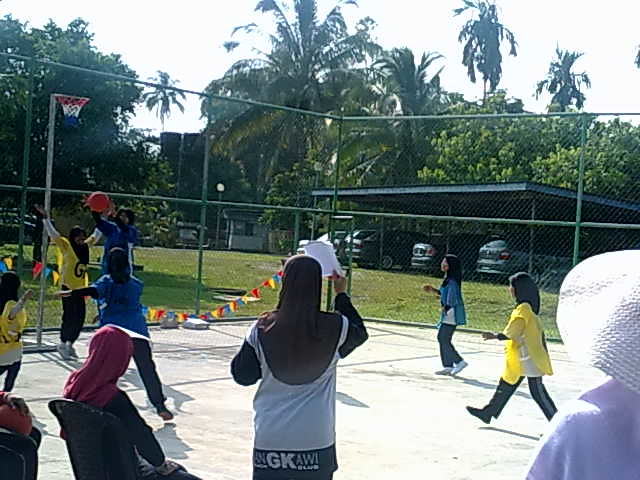The photograph captures an outdoor public basketball court, where a group of women, all wearing black veils over their heads but not covering their faces, are actively engaged in a basketball game. The players are divided into two teams, one wearing yellow uniforms and the other blue. On the left side of the image, a player in blue is holding the ball while a yellow-uniformed player tries to block her with raised arms. 

In the foreground, several women are either seated or standing, with one standing figure waving a piece of paper, possibly a coach or an organizer. They, too, are wearing veils. In the bottom right corner, a spectator in a white brimmed hat can be seen watching the game. Beyond the chain-link fence that surrounds the court, there's a carport with four parked cars. The scenery includes some palm trees, a large expanse of grass, and a white sky, adding to the atmosphere of a sunny day in an open, spacious area. A red, white, and blue basketball hoop is prominently displayed as part of the court setup.